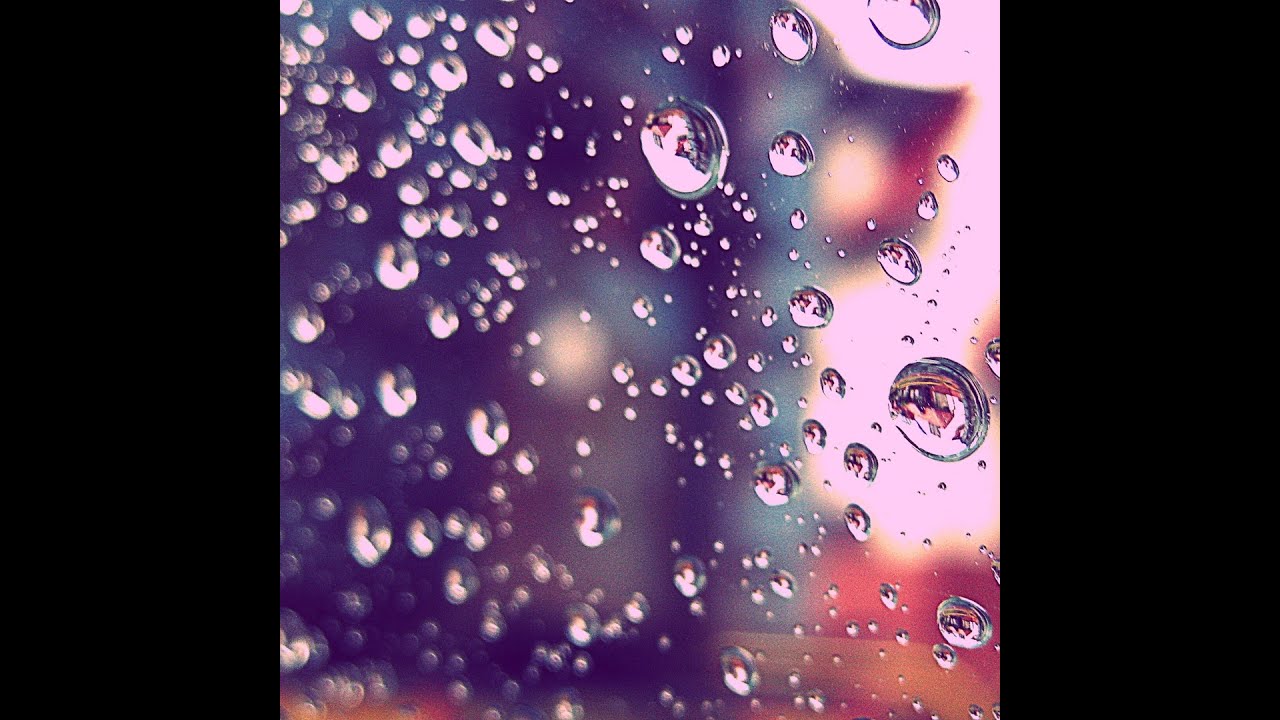The close-up image captures a mesmerizing collection of raindrops scattered across a clear glass window, framed by wide black vertical bars on either side. The scene is mostly bathed in a dark blue hue, gradually transitioning to a blend of yellow and rose tones on the right, adding a touch of warmth and vibrancy. The background is an indistinct, blurry outdoor environment, heightening the focus on the raindrops themselves. The droplets vary in size, with some larger droplets predominantly on the right side, while countless smaller ones are dispersed throughout. Each raindrop mirrors its surroundings, creating tiny, inverted reflections of a distant house with a visible roof and perhaps chimneys, intricately detailed despite their minuscule scale. The focus subtly shifts across the image, with the droplets on the right being sharply defined, contrasting with the progressively blurred ones on the left and towards the bottom. The composition as a whole presents an enchanting snapshot of a rainy moment, beautifully framed and richly detailed.